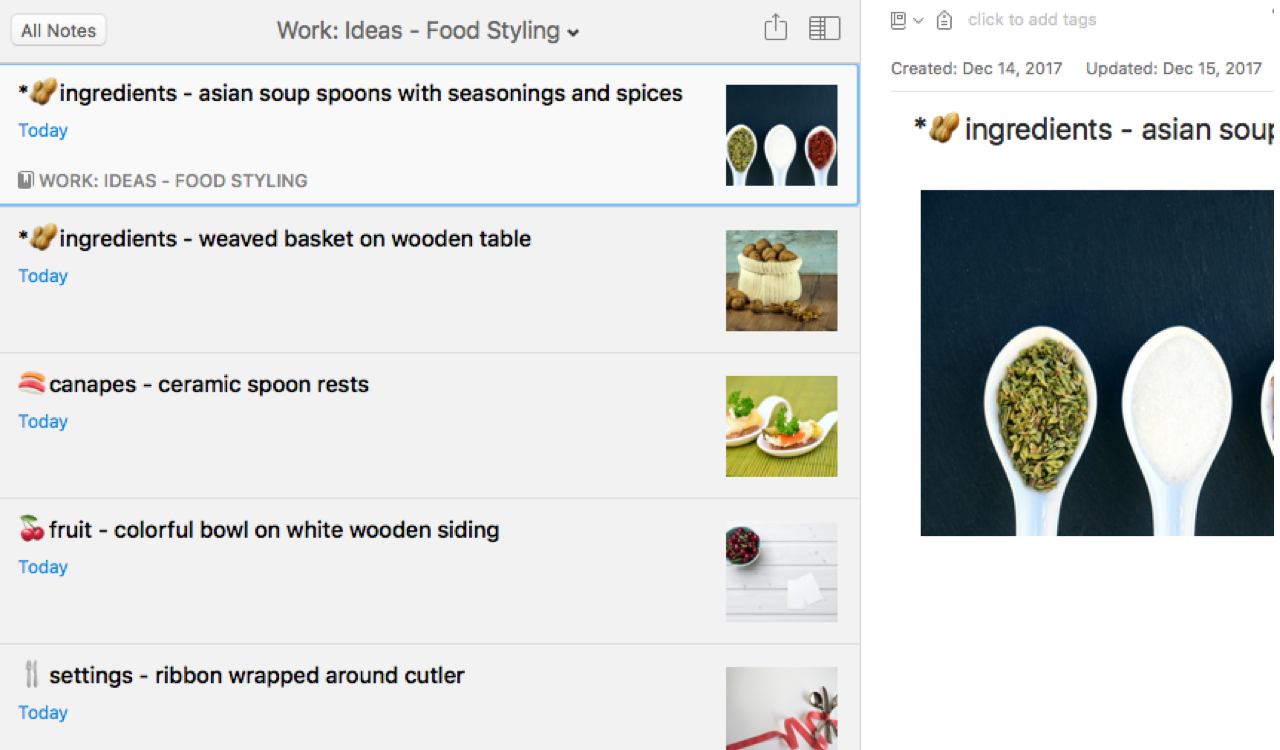The image features a meticulously arranged scene against a white background, dominated by a gray rectangle inscribed with the words "Work Ideas" and "Food Styling" in black text. Various ingredients and props are artfully displayed, including Asian soup spoons filled with a variety of seasonings and spices. 

A woven basket rests on a wooden table alongside a bag of potatoes and an elegant assortment of canapés. Ceramic spoon rests and a ribbon-wrapped cutlery setup accompany a colorful bowl of fruit, possibly cranberries or cherries, placed atop white wooden siding. The phrase "Today" appears multiple times in a distinct blue font. 

Additionally, the caption notes the image was created on December 14, 2017, and updated on December 15, 2017, with these details enclosed in a blue square at the right edge of the image. The composition also includes three white wooden spoons prominently positioned in the foreground.